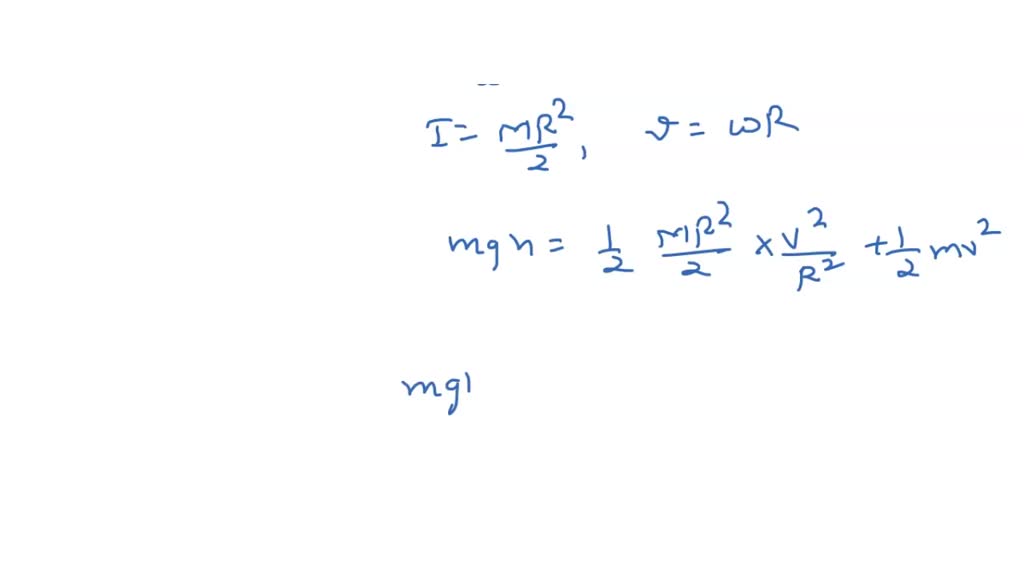This photograph captures a handwritten set of mathematical equations scribbled in blue ink on a white background. The equations, written somewhat messily, span three lines and read as follows: "I = MR² / 2," "T = WR," "MGH = 1/2 MR² / 2 * V² / R² + 1/2 MV²," and at the bottom, slightly outdented to the left, "MGL." The equations appear to be related to physics or engineering, though their exact meanings may be elusive to a layperson. The dark blue ink contrasts sharply with the white background, making the handwritten text stand out prominently.